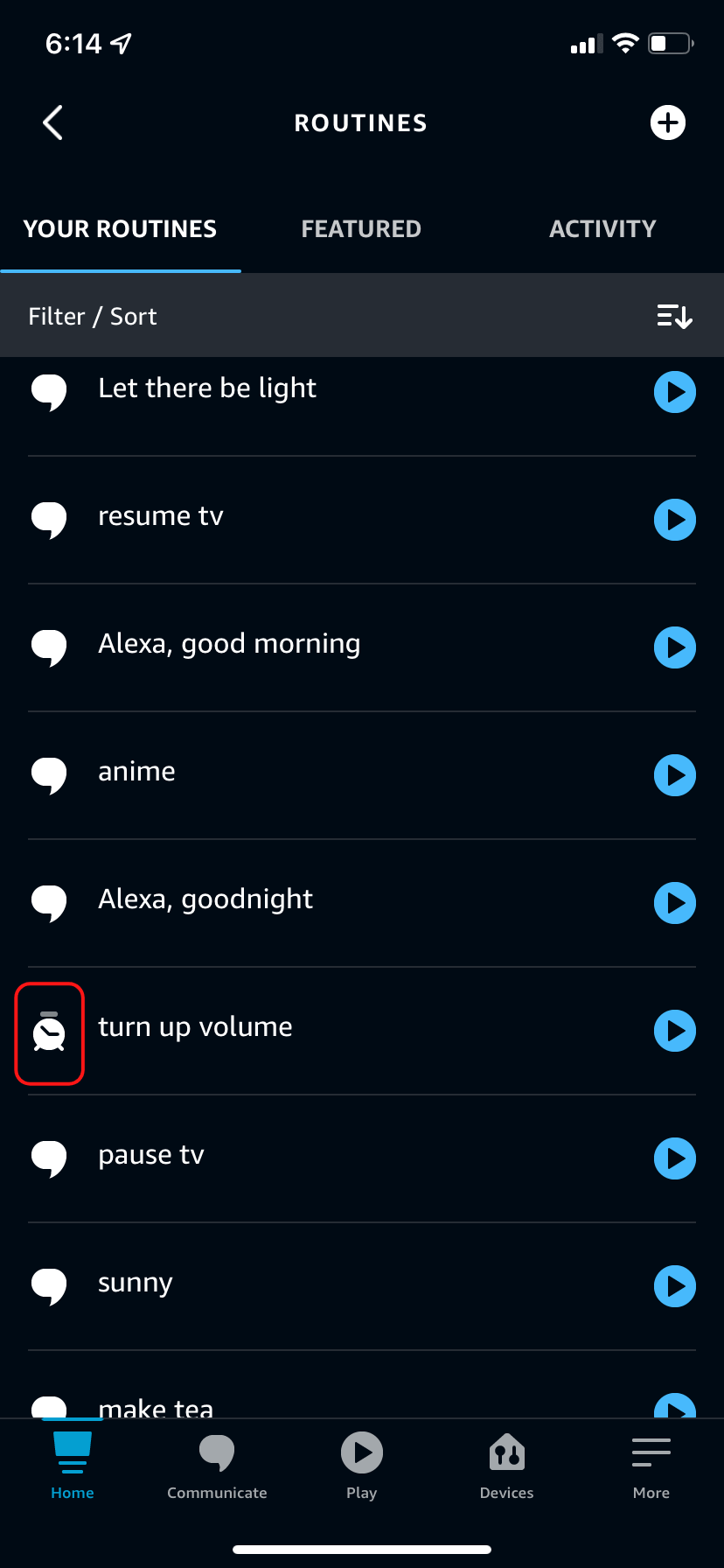Here is a detailed and cleaned-up caption for the image described:

---

The screenshot, taken on a smartphone, displays the "Routines" tab within an app. At the top of the screen, the status bar shows the time as 6:14, with an arrow pointing northeast. Signal strength indicators show two bars, a fully connected Wi-Fi symbol, and the battery is slightly under half full. "Routines" is prominently displayed beneath the status bar, with a back caret on the left and a plus sign on the right. 

The "Routines" tab is underlined in blue, indicating it as the current selection among three available tabs. There's a filter or sort option visible, followed by a list of various routines, possibly related to music or media control. Each routine has a blue circle with a play icon to its right, indicating that they can be activated.

The listed routines include:
- Therapy Light
- Resume TV
- Alexa, Good Morning
- Anime
- Alexa, Goodnight
- Turn Up the Volume
- Pause TV
- Sunny
- Make Tea (partially cut off at the bottom of the screen)

A red box highlights the "Turn Up the Volume" routine, which also has an alarm clock icon to its left, differing from the conversation bubble icons next to the other routines. 

At the bottom of the screen, typical phone navigation options are visible, including "Home," "Communicate," "Play," "Devices," and "More."

---